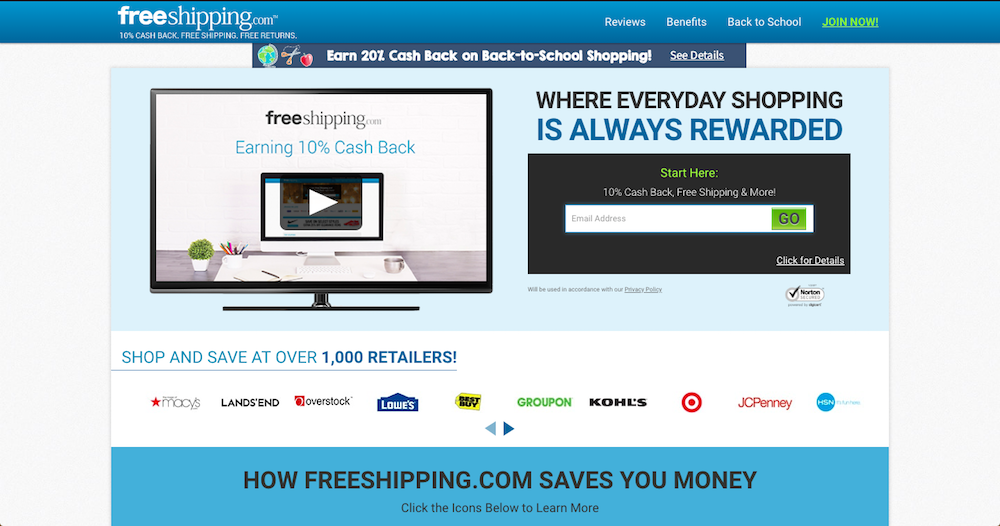The webpage for freeshipping.com features a detailed layout with a light gray background. A prominent blue banner stretches across the top from left to right, displaying white text. In the upper left corner, the banner reads "freeshipping.com" followed by "10% Cashback," "Free Shipping," and "Free Returns." Towards the middle right of the banner, the options for "Reviews," "Benefits," and "Back to School" are listed. There is also an inviting "Join Now" option in green, underlined text.

Centrally positioned beneath this is a smaller, darker gray banner with white text, adorned with icons of a globe, a pair of scissors, and a red apple. The banner proclaims, "Earn 20% Cashback on Back to School Shopping - See Details."

Immediately below this banner sits a computer monitor with a black outline and stand, displaying a primarily white background. The text on the monitor reads "freeshipping.com" in black, followed by "Earning 10% Cashback" in blue. Below this text is a play button for a video. Adjacent to the monitor, black text declares, "Where everyday shopping" with blue text underneath completing the phrase "is always rewarded."

Beneath this section, there is a black rectangle with the phrase "Start here" in green text. In white text, it advertises "10% Cashback, Free Shipping, and More." Accompanying this is a bar to input an email address and a green "Go" button. Below that, more white text urges visitors to "Click for details."

At the bottom of the page, it showcases a list of retailers where shoppers can save, including Macy's, Lands' End, Overstock, Lowe's, Best Buy, Groupon, Kohl's, Target, JCPenney, and the Home Shopping Network.